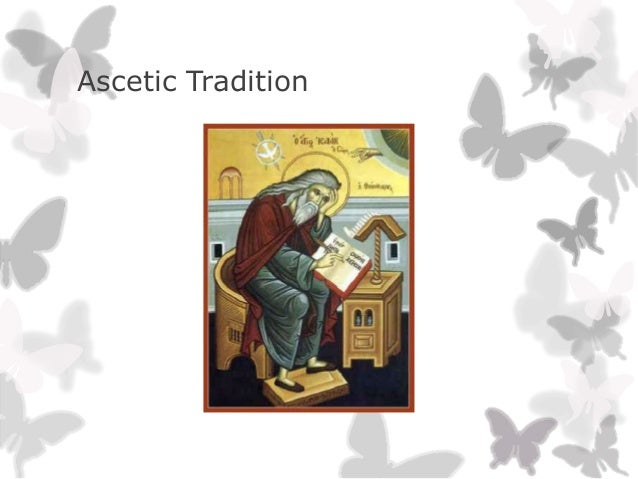The book cover features a solid white background adorned with numerous gray and light gray butterfly silhouettes flanking both sides. These butterflies cascade down the left and right edges, merging toward the center at the bottom. In the upper left corner, in black text, the title reads "Ascetic Tradition," left-aligned. Centrally positioned within this butterfly-accented border is a vertically aligned rectangular image that vividly depicts a saintly figure. This saint, portrayed with long white hair, a beard, and a red robe layered over what appears to be dark gray or blue garments, is engrossed in writing in a book while seated at a wooden desk. His sandals rest on a small wooden platform below the desk. Additional details include a side table with a lamp bearing an upside-down V-shaped shade, a gray and yellow background, and a halo encircling the saint’s head. There's also a diving dove and a hand emanating from a sun motif in the upper right corner. The overall aesthetic suggests a medieval or religious theme, highlighting the saint’s serenity and scholarly focus.